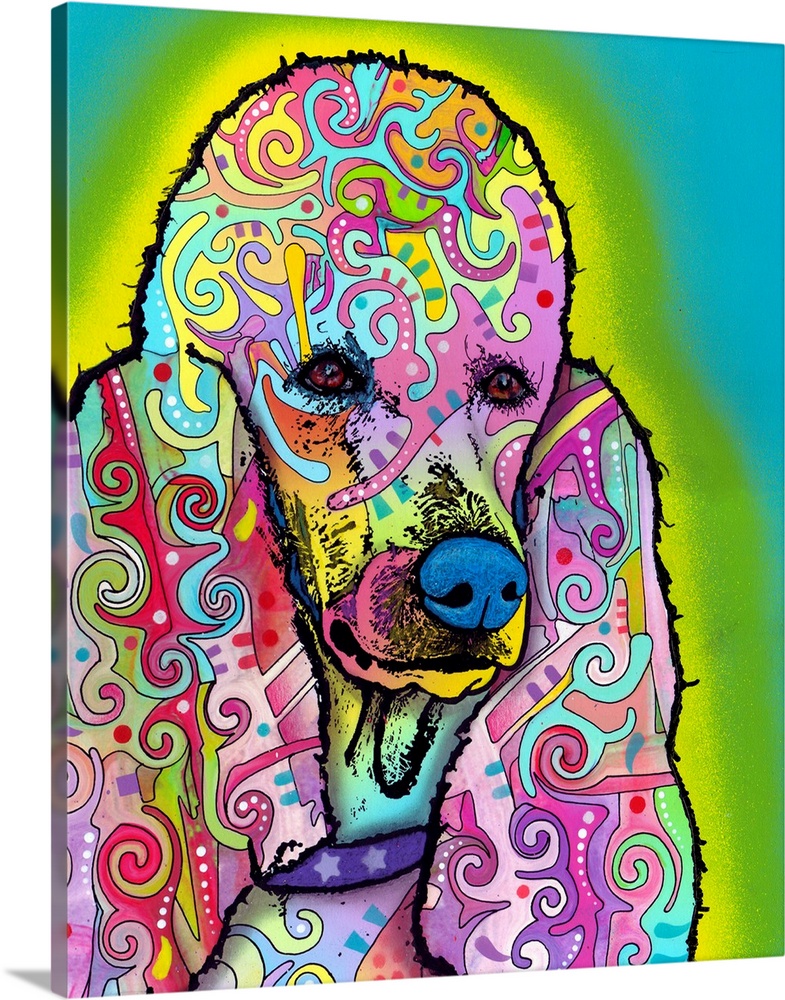This vibrant and surreal artwork features a poodle, filling the entire canvas with its vividly detailed face and fur. The piece, appearing digitally rendered but reminiscent of a psychedelic print or modern art painting, is brimming with a spectrum of flamboyant colors including pinks, purples, blues, yellows, and greens. The poodle's fur is adorned with intricate, swirling patterns, akin to those found on an old psychedelic band's album cover, with amoeba-like shapes, dots, and paisley-esque designs creating a kaleidoscope effect.

The poodle's facial features—eyes, nose, and mouth—are rendered with realistic proportions and detailed enough to suggest that they might be screen-printed. The eyes are natural-looking, while the nose is strikingly blue. The application of color gives the face a glowing, neon, blacklight appearance, enhancing the surreal, psychedelic vibe. The muzzle is detailed, with black speckled fur near the nose adding to the lifelike depiction.

The ears, large and flat, like those of a traditional poodle, extend from the head, decorated with the same swirling, vibrant patterns as the rest of the fur, contributing to the overall psychedelic aesthetic. Surrounding the poodle is an aura of neon green and yellow with light blue hues in the background, furthering the sense of a glowing, otherworldly presence. The backdrop emphasizes the surreal nature of the painting, ensuring the poodle remains the focal point on what appears to be a rectangular frame set against a white background.